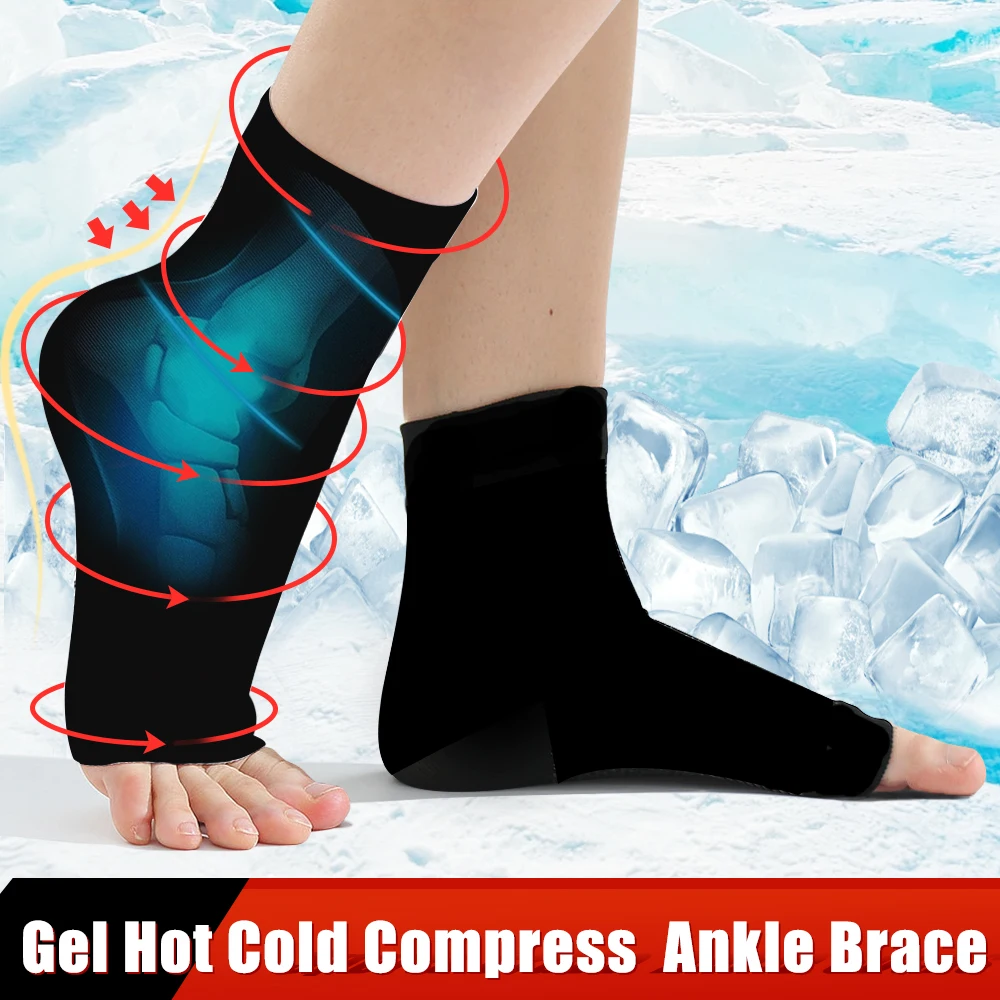This detailed product image showcases the lower legs and feet of a Caucasian female model against a backdrop resembling an arctic region, complete with illustrated ice cubes and snowy terrain to imply a cold environment. The focus is on her feet adorned with black, open-toe ankle braces designed for hot and cold compression therapy. The brace on her left foot extends from just above the ankle to the base of the toes, while the right foot is slightly raised on tiptoe, enhancing the visibility of the brace's supportive structure. Detailed red and blue diagram circles with arrows on the right brace indicate the areas targeted by the thermal features, mimicking an x-ray effect to highlight the ankle bone and joints. At the bottom of the image, a two-toned black and red rectangular banner with white sans-serif text reads "Gel Hot Cold Compress Ankle Brace," marking the image as an advertisement for the product's dual therapeutic functionality.